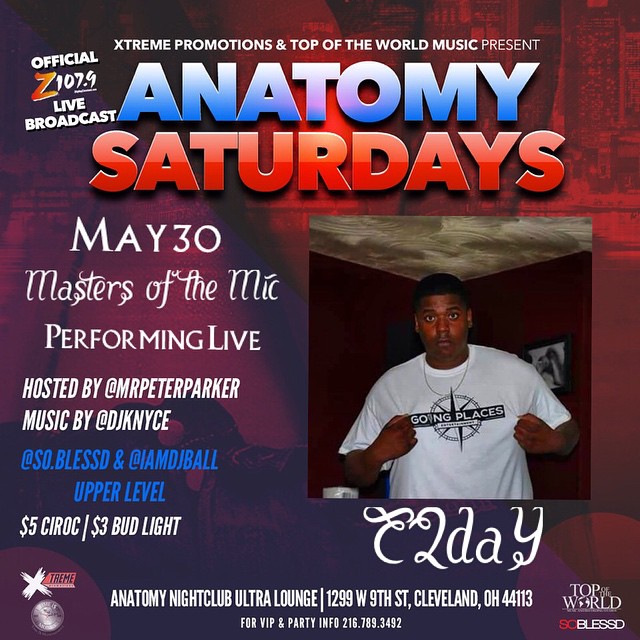The poster features an eclectic blend of vibrantly colored text and clear visual elements to announce a live broadcast event. At the top left corner, the title "Official Z107.9 Live Broadcast" is prominently displayed. Centered at the top, the poster reads "Extreme Promotions and Top of the World Music Presents," highlighting the collaborative efforts behind the event. Below, in large blue and red letters, it boldly announces "Anatomy Saturdays," with "Anthony" in blue and "Saturdays" in red.

Down the left side of the poster, the date is highlighted with much anticipation: "May 30 Master of the Mic Performing Live." The event promises engaging performances hosted by @MrPeterParker, with music spun by @DJKNYCE. Additional musical contributions will feature @SoulBlasted and @IamDJBoo on the upper level. The offerings include $5 CIROC and $3 Bud Light, enticing attendees with affordable drink options.

On the right side of the poster, there is an image of a young Black man wearing a white short-sleeve t-shirt. He is staring directly ahead, with the text "going places" prominently displayed at the center of his chest, symbolizing ambition and forward motion. The combination of striking colors, detailed event information, and engaging visuals makes the poster both informative and eye-catching.